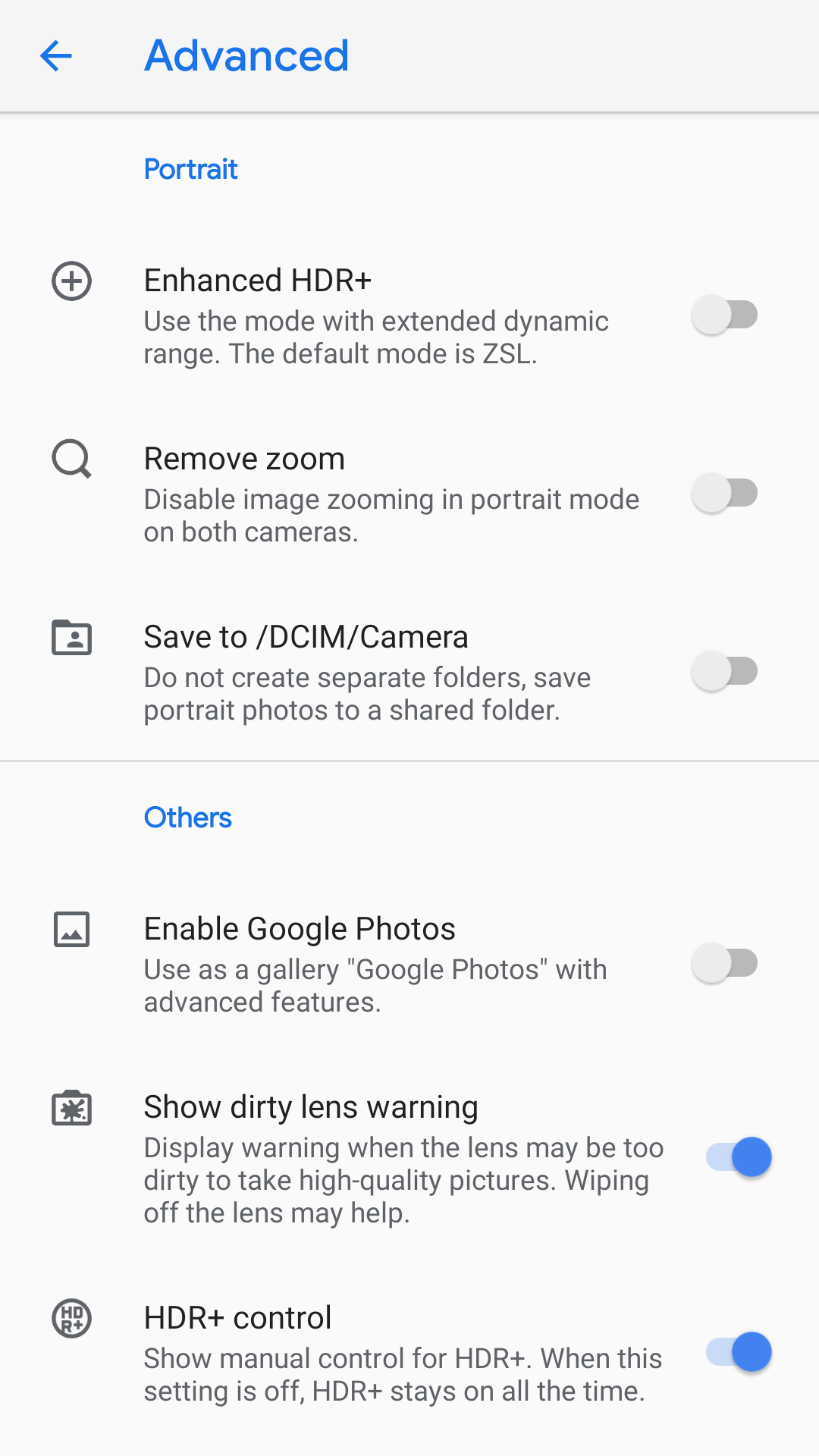**Screen Capture of Advanced Settings Menu: A Detailed Breakdown**

At the top of the captured settings menu, there is a prominent white bar featuring "Advanced" in blue font with a back arrow icon adjacent to it. This indicates navigation is available to return to a previous screen. Below this, the settings are categorized and listed with specific controls and their descriptions.

1. **Portrait Mode Settings:**
   - **Enhanced HDR:** Accompanied by a blue "Portrait" label and a plus sign within a circle, this setting reads, "Use the mode with extended dynamic range." The default mode mentioned here is **ZSL (Zero Shutter Lag)**, which is highlighted by a gray circle.

2. **Image Zoom Settings:**
   - **Remove Zoom:** Next to a gray magnifying glass icon, this option reads, "Disable image zooming in portrait mode on both cameras," with a corresponding gray circle for toggling the setting.

3. **Save Location:**
   - **Save to `/DCIM/Camera`:** Displayed with an icon resembling a manual folder and a small person icon, this directive states, "Do not create separate folders. Save portrait photos to a shared folder," validated by a gray circle.

4. **Other Settings:**
   - **Enable Google Photos:** Beneath the "Others" heading in blue font, there is a depiction of a sheet with mountains, signifying this setting. It reads, "Use Google Photos as a gallery with advanced features," with a gray circle to toggle.
   - **Show Dirty Lens Warning:** Represented by a camera with a starburst dirt icon, this setting states, "Display a warning when the lens may be too dirty to take high-quality pictures. Wiping off the lens may help," paired with a blue circle for activation.
   - **HD + R Control:** The final setting features a small circle icon labeled "HD + R." This reads, "Show manual control for HDR +. When this setting is off, HDR + stays on all the time," marked with another blue circle for activation control.

The detailed breakdown and illustrative icons guide the user through configuring advanced camera settings to optimize functionality and manage photo quality efficiently.